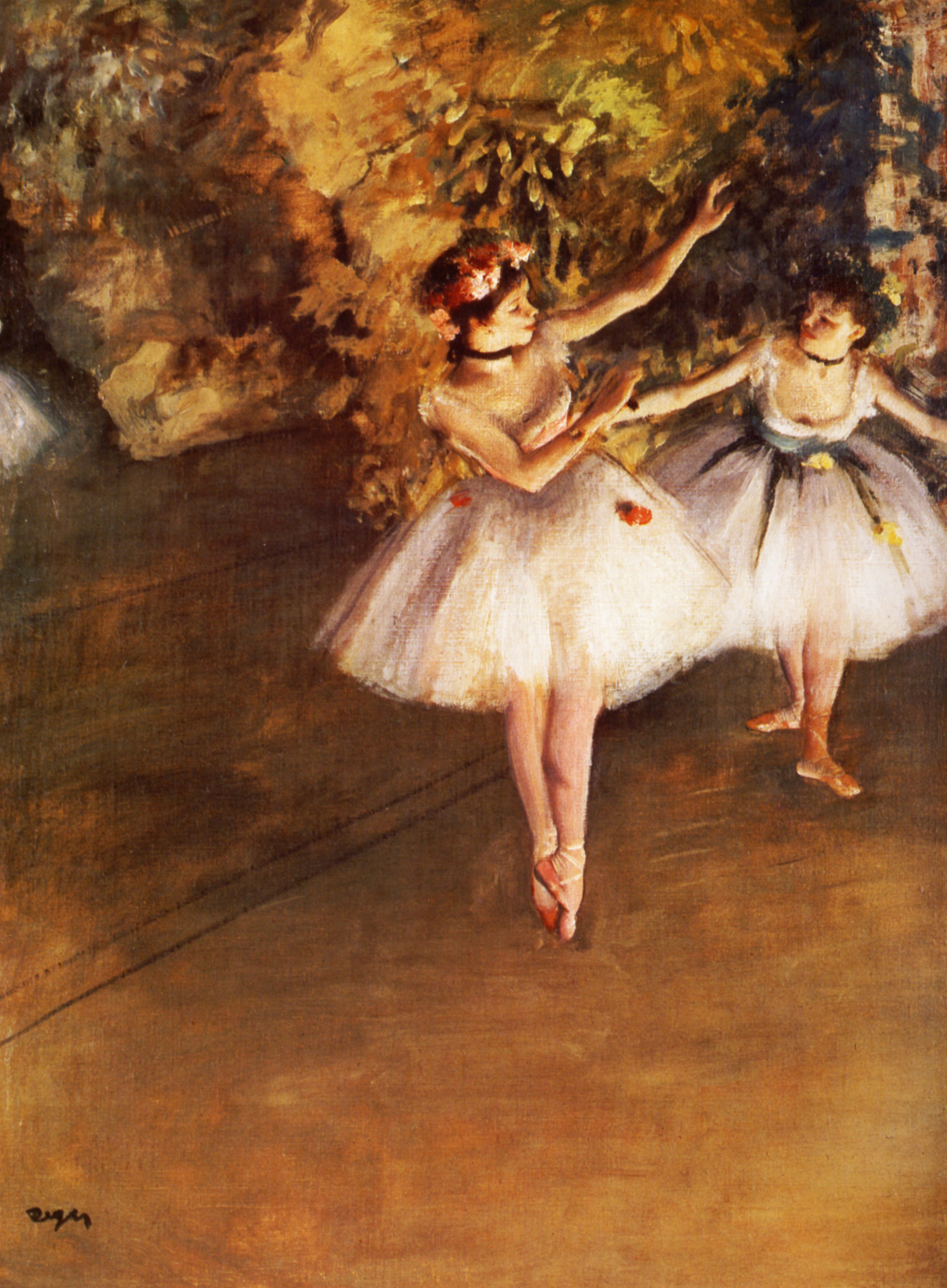The image depicts a detailed and vibrant color painting of two Caucasian ballerinas performing on a light brown, golden-hued wooden stage. Both girls have dark hair and are dressed in similar low-cut, wide-skirted white dresses. The ballerina on the left, who appears taller and stands on her toes, wears red or orange flowers in her hair and matching colored spots on her dress, along with red or orange slippers. Her left arm is gracefully outstretched above her head, while her right arm is bent in front of her torso.

The girl on the right stands flat-footed, with her body oriented towards her dancing partner. She adorns blue and gold flowers in her hair and has a gray band around her waist. Her white dress features two yellow spots. Her arms are extended outward, and she too wears soft ballet slippers. The stage itself extends to a backdrop of textured orange and green hues with an elaborate, feathery gold structure, which might be a decorative element resembling trees.

The artist’s signature is located in the bottom left-hand corner in black, though it is too small to decipher. The background adds depth and context to the ballet scene, enhancing the overall composition of the painting.